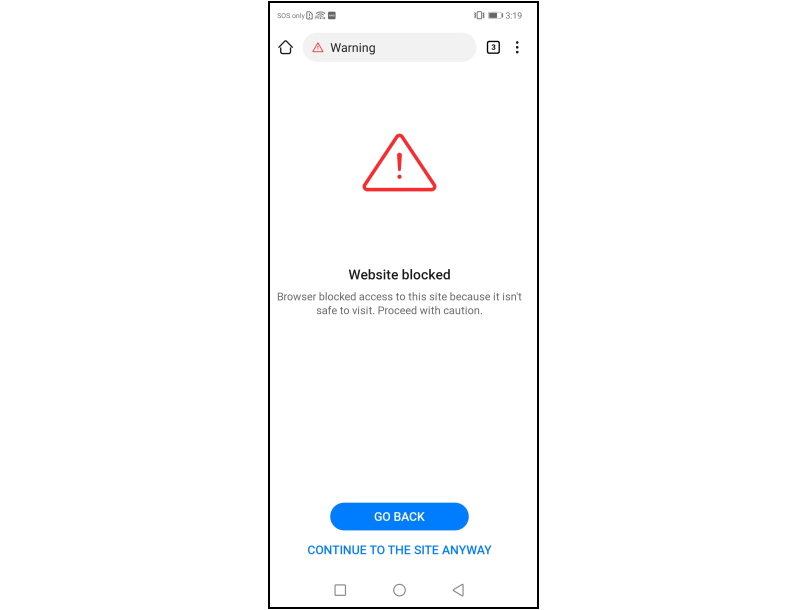This image, captured on a smartphone, depicts a browser warning screen. At the top of the screen, there is a search bar featuring a small triangle tipped with red and containing a red exclamation point, alongside the word "Warning." Below this, the screen shows a much larger red triangle with an exclamation point at its center. The text below the triangle reads: "Website blocked. Your browser has blocked access to this site because it isn't safe to visit. Proceed with caution." 

A significant blank space follows this warning message. Towards the bottom of the screen, a blue button labeled "Go Back" appears, with an additional blue text below it stating, "Continue to the site anyways." 

At the very bottom of the screen, there's a gray footer. This footer contains a gray circle in the middle and a triangle pointing to the left on the right side. The top right corner of the screen shows the time as 3:19 PM, a battery icon indicating roughly two-thirds charge, and additional unidentified icons on the left.